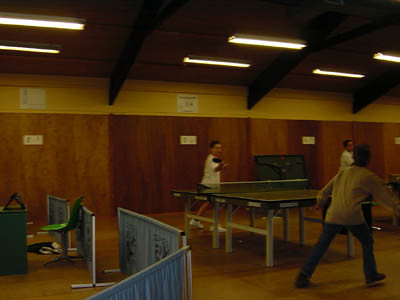This color photograph, taken indoors with noticeably poor lighting, captures a scene dominated by a ping pong match. The room, reminiscent of an old recreational facility, features long, fluorescent strip lights on a dark ceiling, casting a dim, tannish hue across the scene. The walls are predominantly wood-paneled up to three-quarters of their height, with a strip of cream or yellow cement extending to the ceiling. Below, the floor is made of wood. 

In the foreground, two players are intensely engaged in their game. The player on the left is dressed in a tan shirt and blue jeans, while his opponent sports a white t-shirt and shorts, mid-action with a paddle. To the left, a set of blue, hip-height screening panels on white stands form a partial barrier, along with some scattered gear and a chair. Also visible in the room is an array of unused gates or fencing panels leaning against the wall, suggestive of a multi-purpose space. In the background, another player can be seen, further emphasizing the lively atmosphere possibly indicative of a local tournament or recreational event.